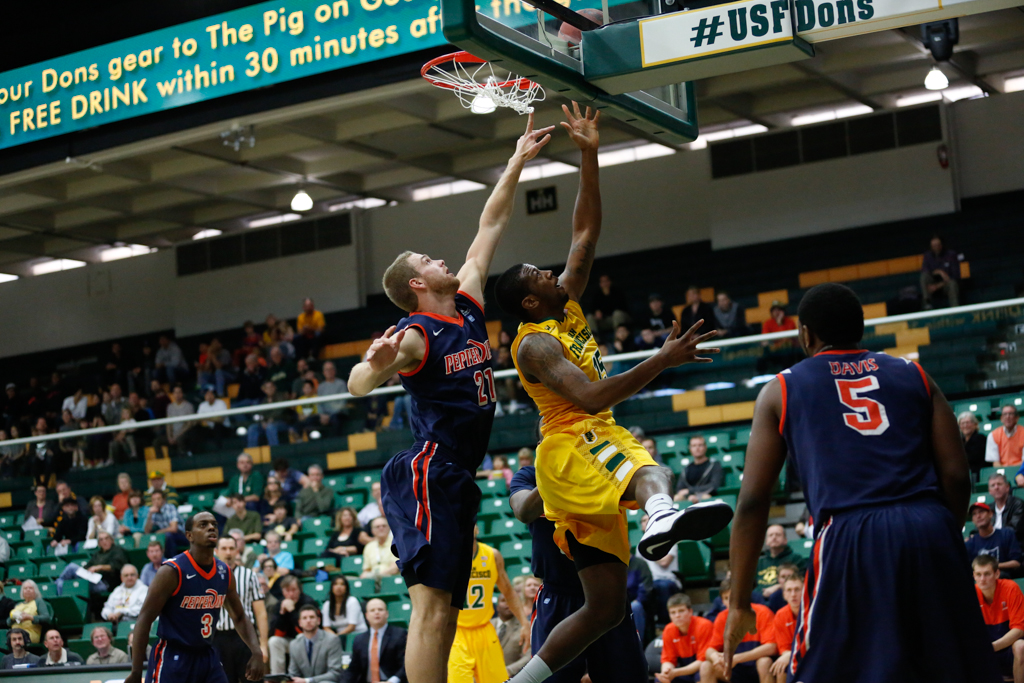In a vibrant, full-color photograph capturing the intensity of an indoor basketball game, multiple players are seen in dynamic action on the court. At the forefront, a player wearing a blue uniform and another in a yellow uniform are leaping towards a clear acrylic backboard with an orange rim and white net, trying to dunk the basketball, while another player attempts to block it. The player in blue is white, and the player in yellow is black. Additional players with jersey numbers 5, 3, 21, and 15 are visible, positioned around the court, with one in the bottom right corner and another in the bottom left.

The setting is a spacious indoor basketball court with a distinct white ceiling featuring multiple square recesses and hanging lights. Behind the court, a large audience fills the bleachers, which are predominantly yellow and green. Despite being vibrant, the stands have pockets of empty seats, suggesting it could be a minor league or small college game. 

Above the action, text can be seen, partially cut off, including the hashtag USFDONS, reference to "Don's gear to the pig," and a sign promising a "free drink within 30 minutes of...". The backdrop wall is white, further illuminating the spirited scene as the audience watches the high-flying action unfold on the court.